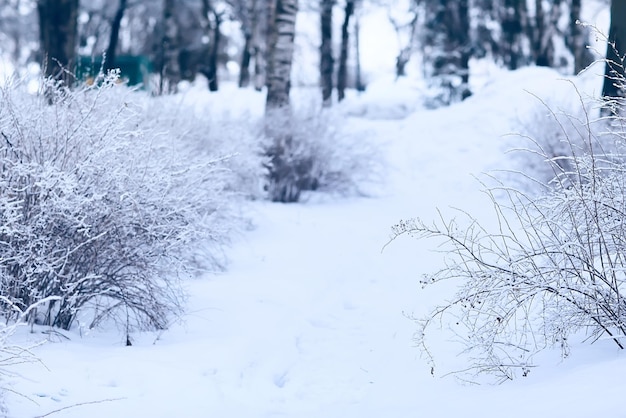This photograph captures a serene winter scene deep within a snowy forest, with a pervasive bluish tint giving the snow an ethereal glow. The foreground features prominent bushes on both the right and left sides, their branches barren yet adorned with a few frozen bulbs or berries. A thick layer of snow blankets the ground and all plant life, enhancing the stark contrast between the white snow and the dark, leafless vegetation. In the distant background, several frosted tree trunks emerge shrouded in a wintry haze, their details blurred to emphasize the closer elements. Towards the top left of the frame, a green, rectangular object—likely a man-made structure, given its painted appearance—adds a touch of contrasting color, with a hint of yellow that could be a sign. This image, rich in detail, beautifully captures the tranquil and desolate essence of a winter forest.